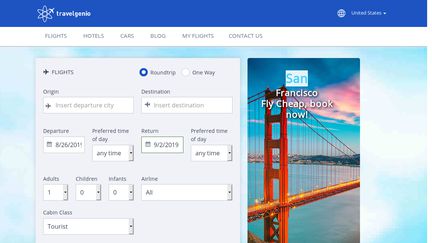The screenshot captures a webpage from a flight scheduling website called "Travel Genie," prominently displayed in the upper left corner against a dark blue background. Beneath the logo, there's a navigation bar with tabs labeled "Flights," "Hotels," "Cars," "Blog," "My Flights," and "Contact Us." 

The lower section of the image features a sky-themed background along the top and side borders, with fluffy blue and white clouds. On the left side, a gray rectangle contains essential flight booking details. It shows that the user has selected a round trip and includes editable fields for "Origin" and "Destination" cities, along with preferences for "Departure Date," "Return Date," "Preferred Time of Day," and more. The specifics are as follows: 
- Departure city: [To be inserted]
- Destination city: [To be inserted]
- Departure Date: [To be inserted]
- Preferred Time of Day: Any Time
- Return Date: 09-02-2019
- Preferred Time of Day: Any Time
- Number of Adults: 1
- Number of Children: 0
- Preferred Airline: All
- Cabin Class: Tourist

To the right of this section, there is an inviting image of the San Francisco Bay Bridge, set against a picturesque backdrop that includes a vibrant sky with a striking pink cloud at sunset. Over this image, there’s promotional text that reads: "San Francisco, Fly Cheap, Book Now."